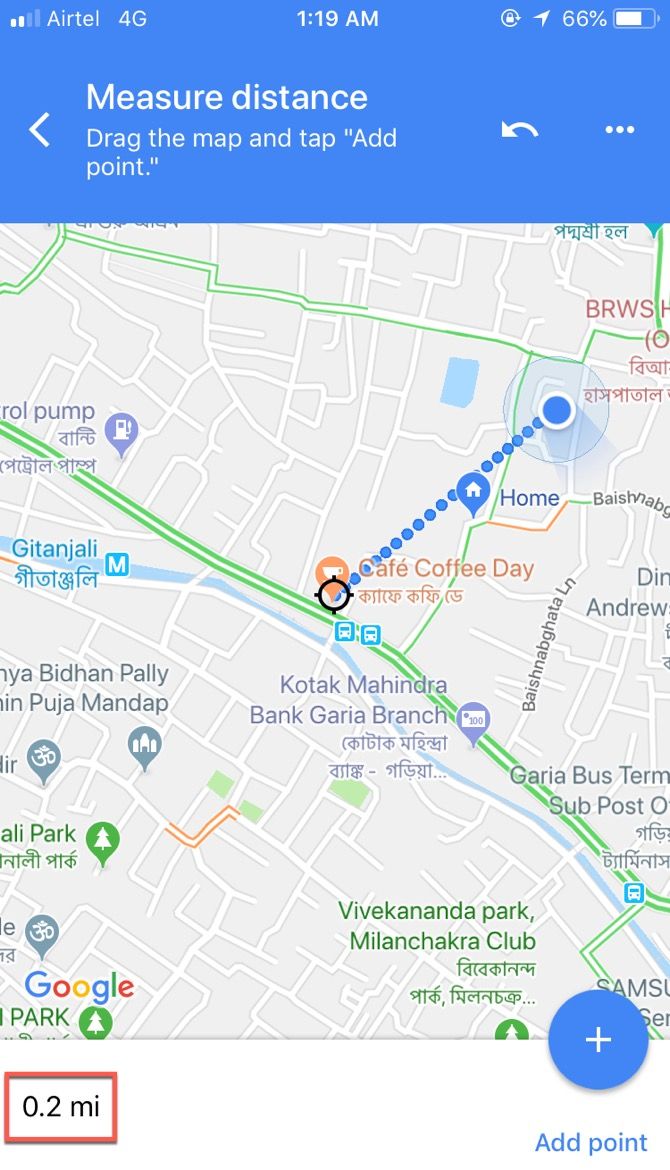The image is a high-resolution, color screenshot of a smartphone displaying a partially visible map application. The screenshot, taken at 1:19 a.m., shows the phone is locked and has a 66% battery charge. The user is connected to the 4G Airtel network, with signal strength indicated as two out of four bars. The map app appears with a light blue banner at the top, different from the familiar Google Maps interface, suggesting it may be Bing Maps or another less common navigation tool.

In the app, there is a measuring tool activated that instructs the user to "Measure distance. Drag the map and tap to add point." The map indicates the user's current location and the target location, identified as Cafe Coffee Day, which is 0.2 miles away. The surroundings on the map hint that the location is in India, with landmarks such as Kotech Mahindra and Vivekananda Park marked nearby. The map's user interface and the distance measurement tool imply that the user is trying to determine the straight-line (as-the-crow-flies) distance between their current position and the destination.